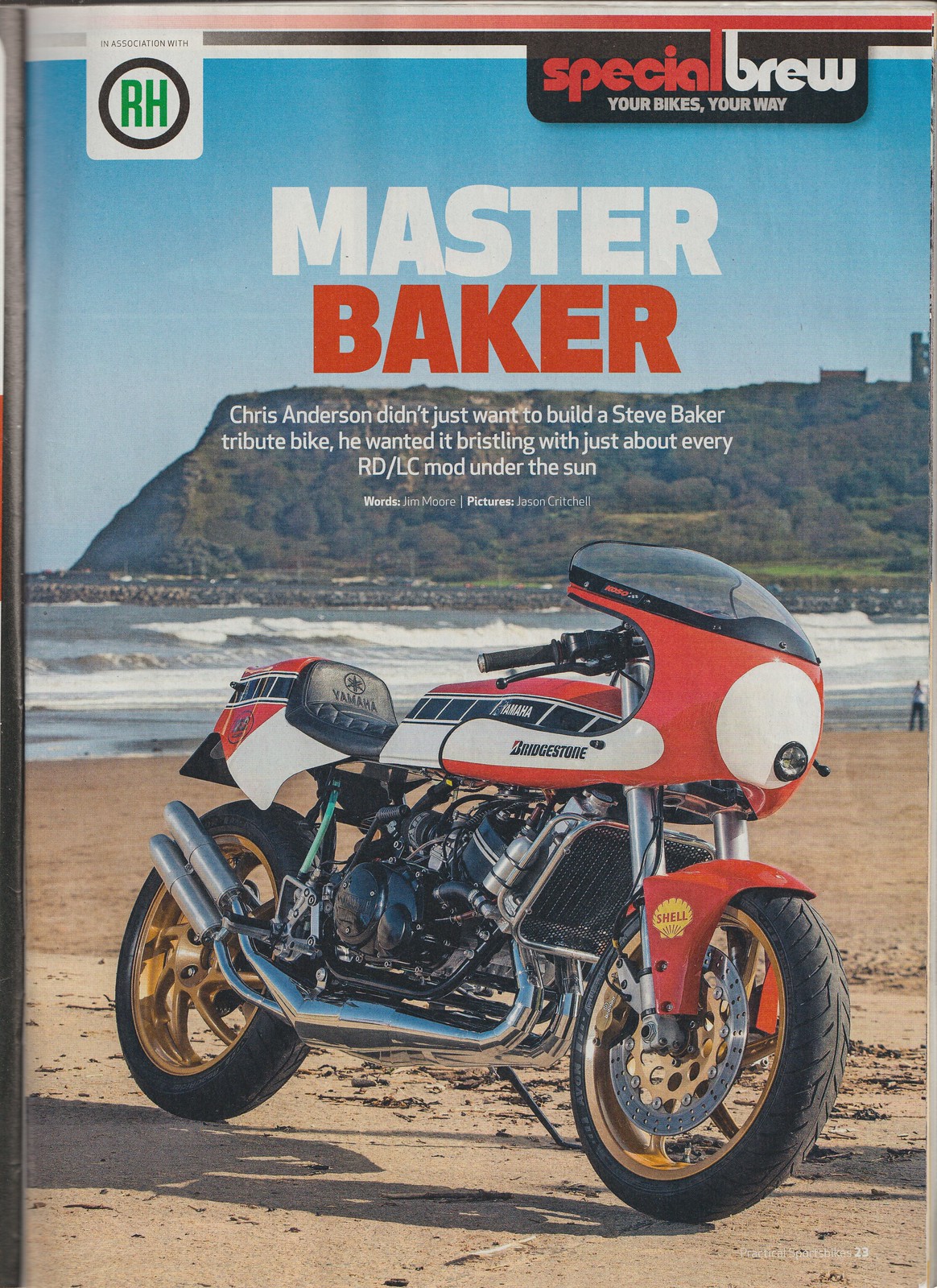This image is an old magazine cover, likely titled "Special Brew: Your Bikes, Your Way." The cover features a bold subheading in white text that reads, "Chris Anderson didn't just want to build a Steve Baker tribute bike; he wanted it bristling with just about every RD/LC mod under the sun." This text describes the focus of the main article or feature, suggesting a deep dive into a custom bike project honoring Steve Baker.

The central image dominating the cover is a striking red and white motorcycle, parked with its kickstand out on a sandy beach. In the backdrop, waves are crashing against the shore, and a lush green mountain forms an impressive silhouette across the horizon. There is also a figure, a man in a blue shirt, standing near the water's edge, enhancing the scene's serene yet adventurous vibe. The magazine may also be associated with the name "Master Baker," which appears prominently below the main title, creating an additional layer of branding or focus on the featured article.